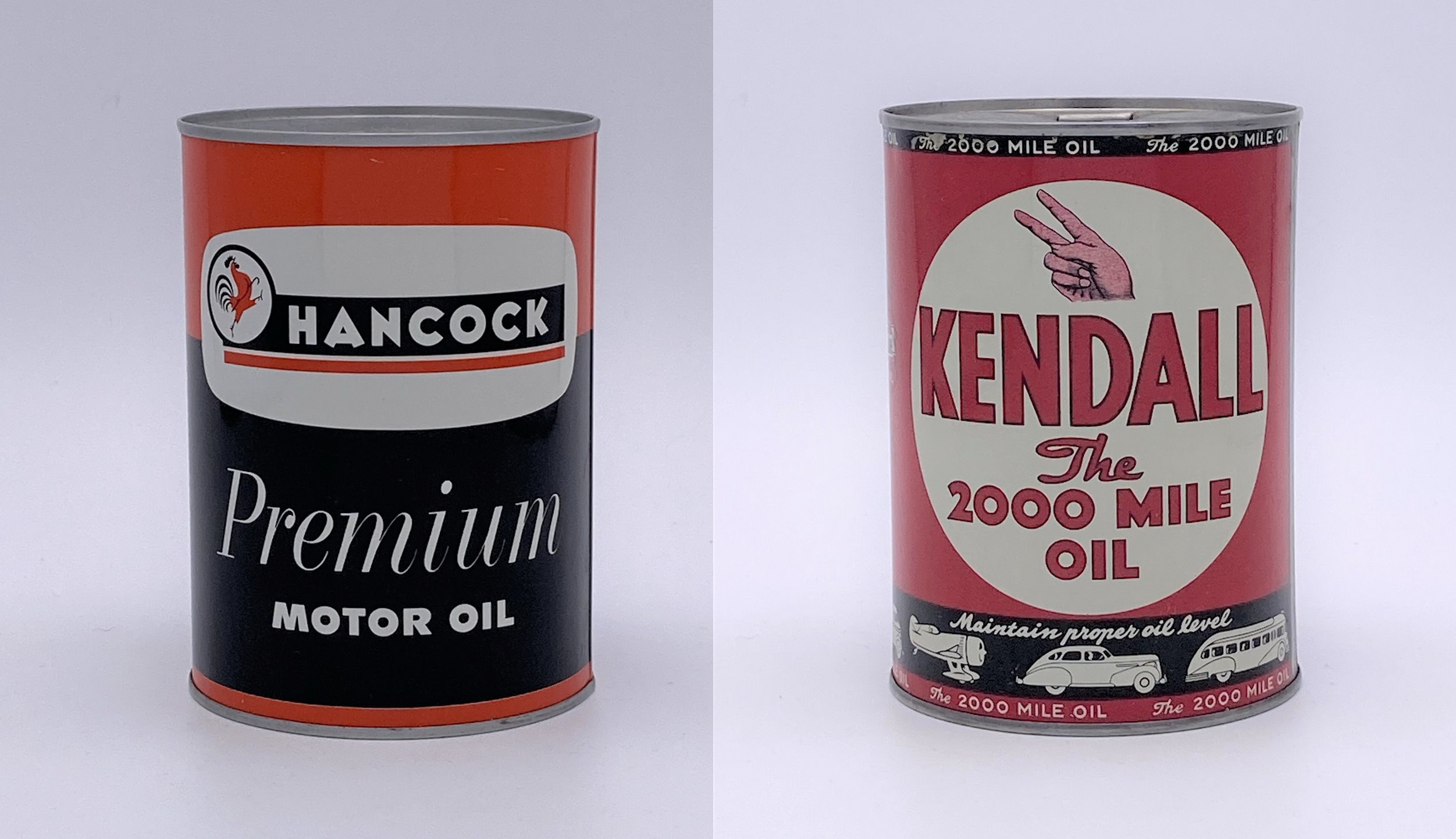This detailed image showcases two retro motor oil cans, displayed side by side in a collage-like format against different shaded backgrounds—one slightly off-white grayish, the other almost white. The left can, a Hancock premium motor oil can, employs an old-fashioned design with red at the top and black at the bottom. The prominent text "Hancock" is accompanied by a prancing rooster logo, followed by "premium motor oil" in a large central font. The right-hand can, branded "Kendall," features the text "2,000-mile oil" and displays an intricate design with a red and black color scheme. This can includes a hand making a peace symbol, with additional text instructing to "maintain proper oil level" and depicting detailed line drawings of a car, bus, and biplane. Both cans evoke a nostalgic vibe of vintage motor oil packaging, standing as historic relics positioned next to each other.